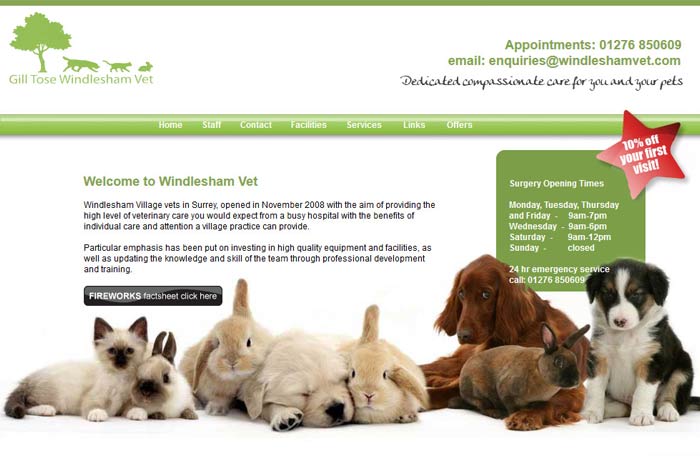The website image features the homepage of Giltos Windlassham Vet. In the upper left corner, nestled within the top banner above a horizontal menu, the clinic's name, "Giltos Windlassham Vet," is prominently displayed in green font. Directly above this, the logo showcases green silhouettes of a tree, a dog, a cat, and a rabbit.

To the right, the banner provides essential contact information with the call-to-action "Appointments." Below this, a contact number is listed, followed by an email address: inquiries@windlasshamvet.com.

Just beneath the banner, a heartfelt tagline reads: "Dedicated, compassionate care for you and your pets." Immediately below this tagline is the website's navigation menu, seamlessly leading to other sections of the site.

Dominating the central portion of the page is a picturesque image of dogs, rabbits, and cats, lending a warm, inviting feel. Above this image, a notice highlights the surgery's opening times. Lastly, a star-shaped graphic announces a special offer: "10% off your first visit."